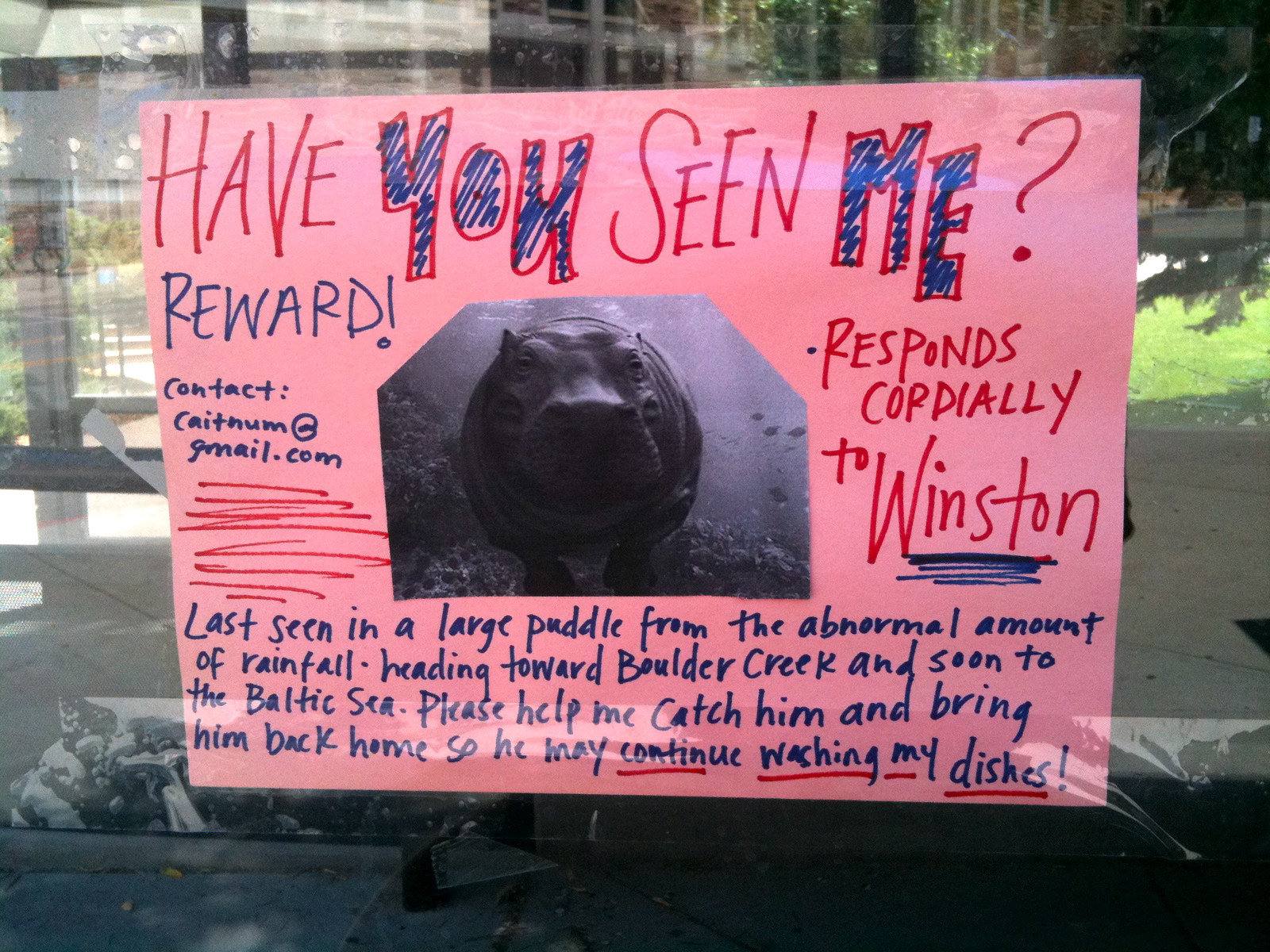The image displays a handwritten, humorously designed pink poster affixed to a window, gleaming with sun reflections. The sign features red and blue text and a black-and-white drawing of a hippopotamus centered on the poster. Boldly at the top, it reads, "Have you seen me?" Below this, to the left, it says, "Reward. Contact Catenum at gmail.com," while to the right of the picture it states, "Responds cordially to Winston." At the bottom, an elaborate narrative reads, "Last seen in a large puddle from the abnormal amount of rainfall heading toward Boulder Creek and soon to the Baltic Sea. Please help me catch him and bring him back home so he may continue washing my dishes!" This poster, likely drawn with crayons or colored pencils, showcases a quirky plea for the return of a lost hippopotamus, with additional whimsical touches evident from the amusing context and intricate layout.